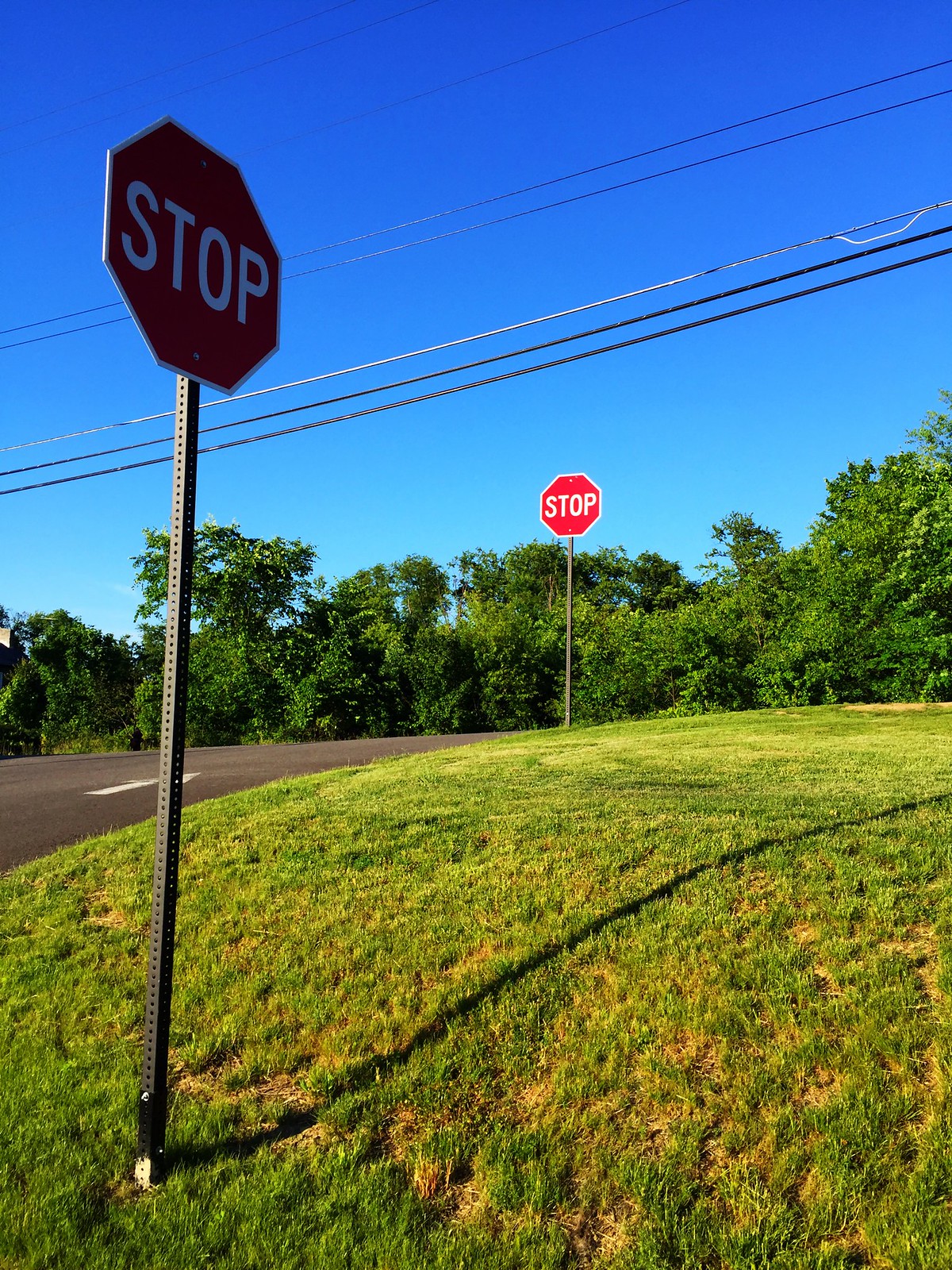In this image, two stop signs are prominently featured within a grassy area under a clear, blue sky with no clouds. The foreground showcases a stop sign mounted on a dark metal pole, positioned so close to the camera that the road is not visible. This stop sign, with its red octagon shape and white lettering, casts a noticeable shadow onto the green grass below. Moving into the distance, there is a slight uphill slope from which another stop sign emerges at the edge of a faintly visible road that enters from the left of the image. This secondary stop sign is shot directly in the center of the frame. Between the two stop signs, various power and telephone lines run diagonally across the sky from right to left. The landscape is completed by a backdrop of dense, green trees spanning the width of the image, which contrasts vividly with the gradient blue sky that deepens in color from horizon to apex. The entire scene is lit by the bright sunlight, illuminating the grass, enhancing the colors, and casting defining shadows.